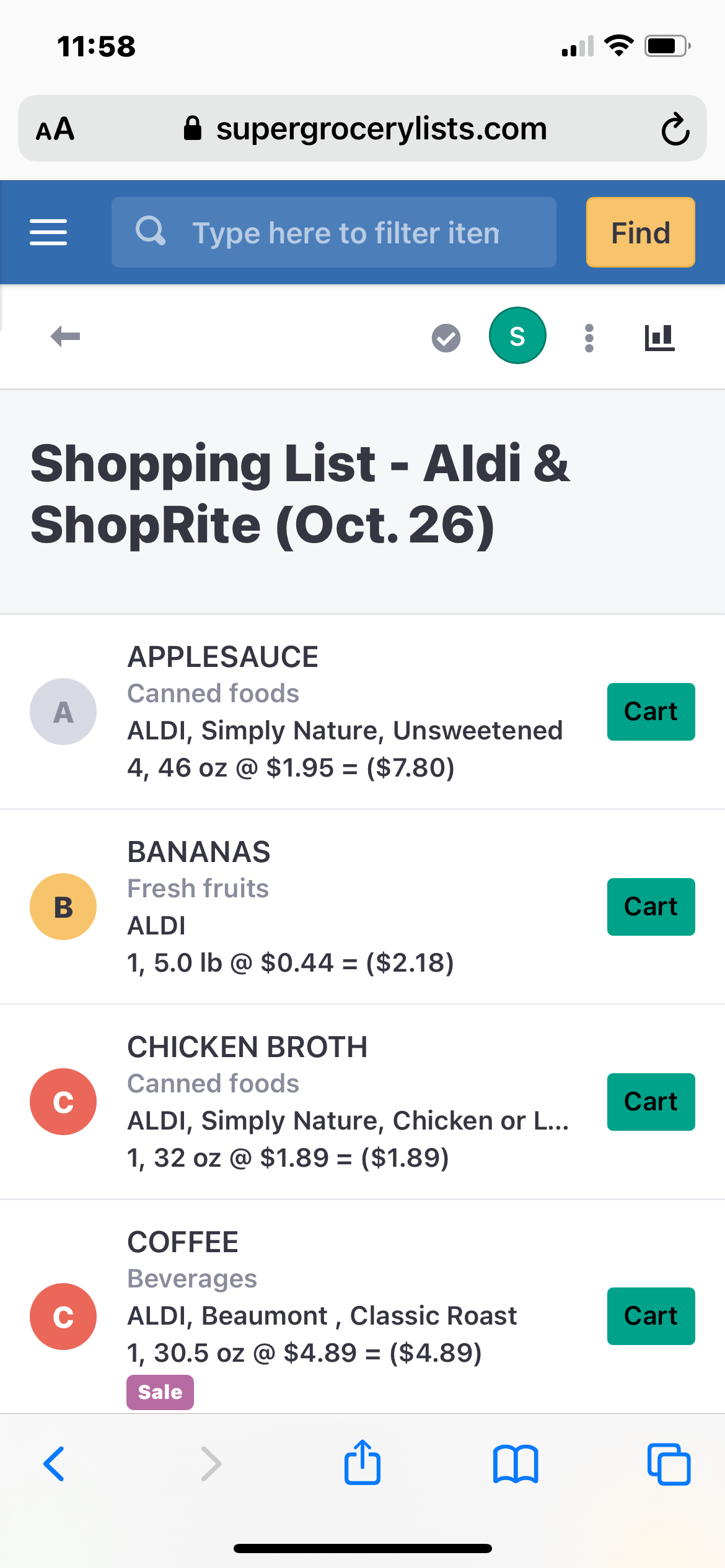This is a detailed, cleaned-up descriptive caption for the provided image narrative:

---

The screenshot captures the interface of a smartphone displaying a web page from SuperGroceryLists.com at 11:58. The smartphone's battery and Wi-Fi signals are both strong. Positioned at the top is a search bar labeled "Type here to filter items," accompanied by a left-facing arrow on the left, a check mark to its right, a white "S" inside a green circle, and three vertical gray dots. Below this header lies a section headlined "Shopping List: Aldi and ShopRite, October 26th," followed by a list of grocery entries denoted by the letters ABCD to the left.

The first entry lists:
- Applesauce, Canned Foods, Aldi, Simple Nature, unsweetened, 46 ounces at $1.95 each, totaling $7.80, featuring a cart button.

The second entry details:
- Bananas, Fresh Fruits, Aldi, 5.05 pounds at $0.44 per pound, totaling $2.18, with an accompanying cart button.

The third entry describes:
- Chicken Broth, Canned Foods, Aldi, Simple Nature, Chicken, 32 ounces at $1.89 each, totaling $1.89, including a cart button.

The fourth entry features:
- Coffee, Beverages, Aldi, Beaumont Classic Roast, 30.5 ounces at $4.89 each, totaling $4.89, marked as on sale, and includes a cart button.

At the bottom of the screen are user interface icons: a blue left-facing arrow, a gray right-facing arrow, a download icon, a bookmark icon, and a lower screen/page icon.